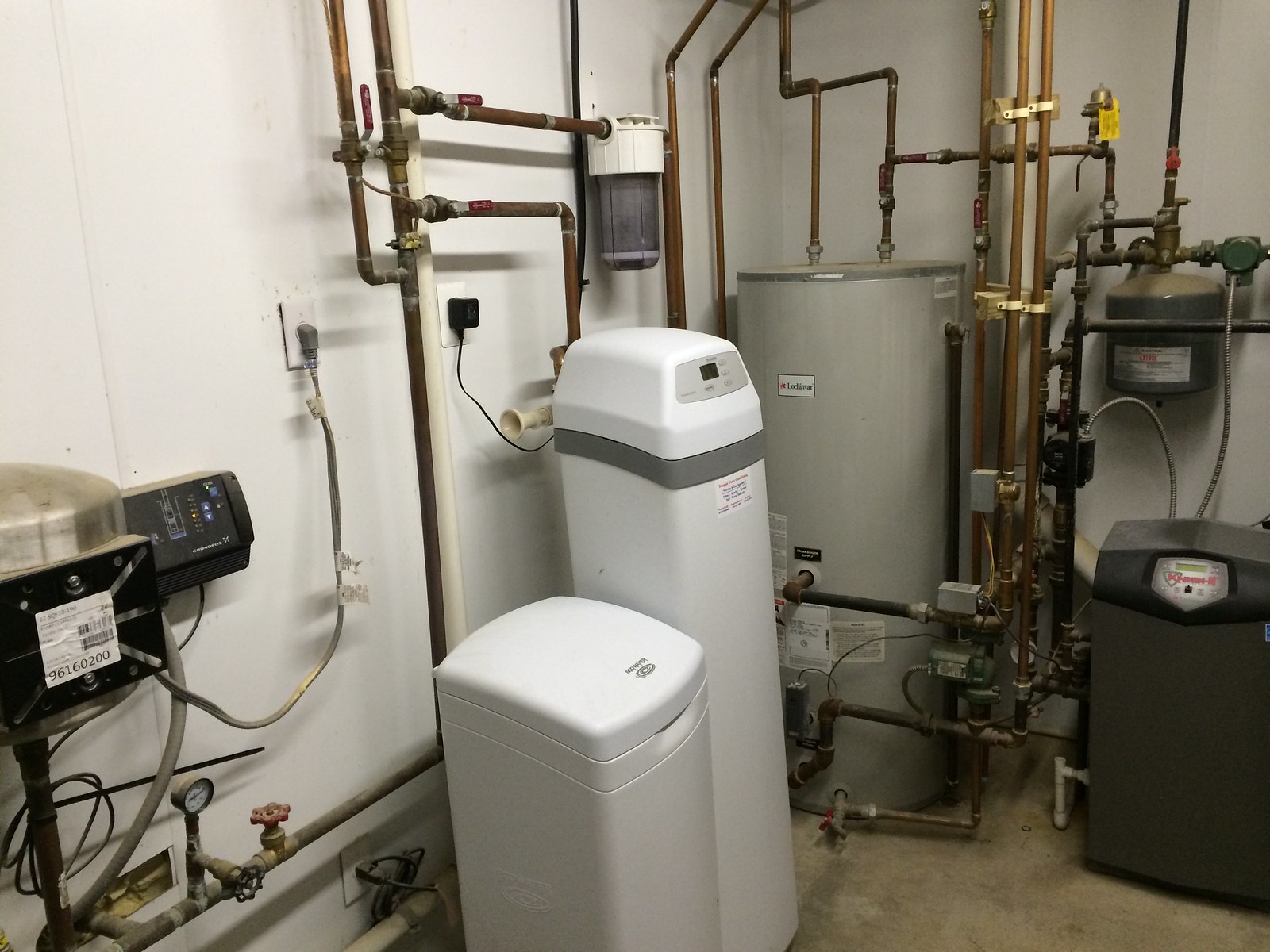This color photo captures an assortment of equipment, likely situated in a garage or basement, with two white-painted walls meeting at a corner and a sandy-colored floor. Dominating the scene is a large, cylindrical hot water heater tank with a distinctive light gray hue, adorned with an intricate network of metal pipes extending from it. These pipes, primarily copper-bronzed, traverse the walls, marked by sharp 90-degree bends and various red and blue stopcock valves. Adjacent to the tank are two white appliances; one looks like a small freezer or trash can with an inconspicuous label, while the other stands taller, featuring a digital display and some printed numbers. In the bottom right, a black machine with grayish-silver coils can be seen, connected to the other equipment through a series of pipes. The overall setup suggests a utility or boiler room filled with complex, interconnected machinery.